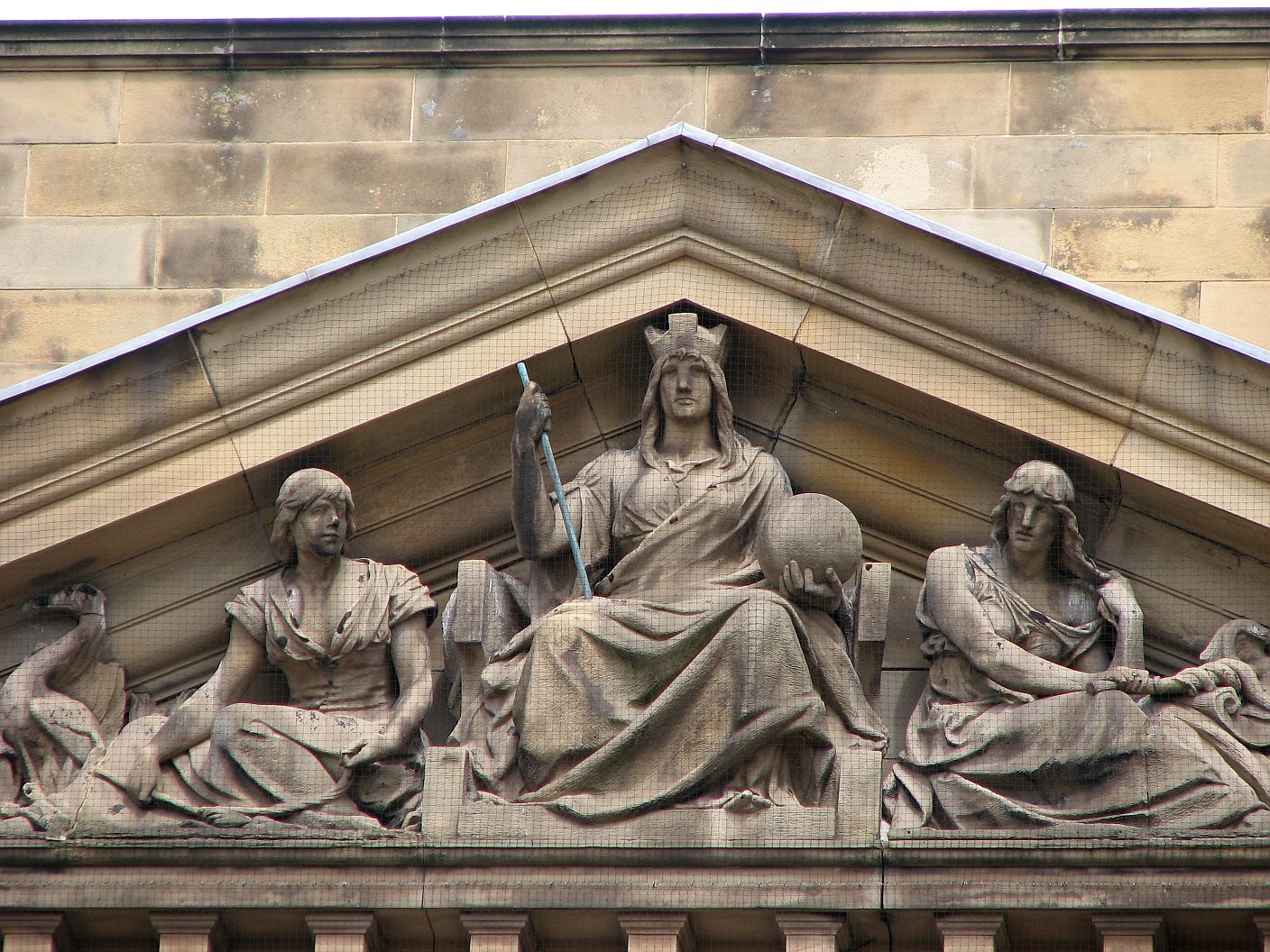The photo captures the top section of a sculpted architectural element, likely the facade of a grand building, featuring three stone statues set within an archway. At the center sits a robed man on a low throne, barefoot, with his toes extending over the edge. He is crowned and holds a staff or rod in his right hand and an orb in his left. The central figure, who appears to be Caucasian with long hair, is flanked by two figures. To his left (the viewer's right), a woman in a long dress is depicted with a smock and a bird—possibly a goose—beside her. On his right (the viewer's left), another woman also dressed in a toga-like outfit, potentially with long hair or a hood, sits holding a length of rope. The statues themselves are rendered in a dark tan stone, giving them an aged, antique appearance. The surrounding architecture suggests a grand entrance or significant portico, hinted at by the visible arch but not fully captured in the image.